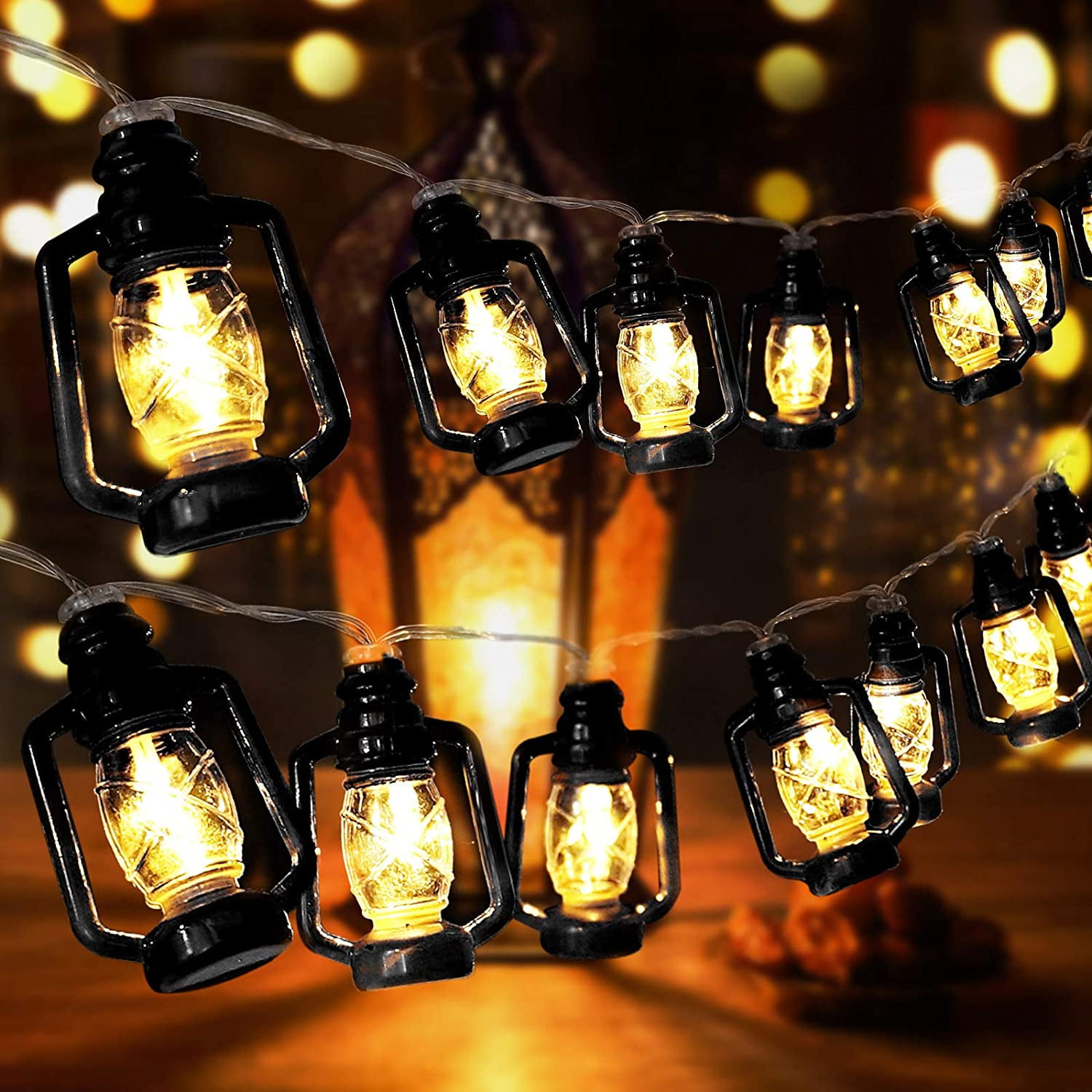This photograph captures an intriguing display of hanging lanterns, meticulously arranged in two rows – six lanterns on the top row and seven on the bottom. Each lantern features a clear, barrel-shaped body illuminated from the inside, accentuated by a framework of black caps and distinctive black handles resembling pitcher handles. The lanterns are suspended by electrical cords, creating a glowing, warm ambiance with their bright yellow light.

In the background, the golden light floor beneath the lanterns adds an extra layer of warmth and charm to the scene. Behind the rows of lanterns, a larger, intricately designed lantern stands out with its frosted panels lit from within, casting a soft, golden glow. The larger lantern appears to be supported by ornate, lazy wrought ironwork, contributing to the ceremonial atmosphere of the setting. Muted ceiling lights complement the overall lighting ensemble, highlighting the detailed craftsmanship of both the lanterns and the surrounding area, which includes an arc or mantel that leads into a darker, less discernible part of the space. This scene exudes a sense of refined artistry and historical ambiance.